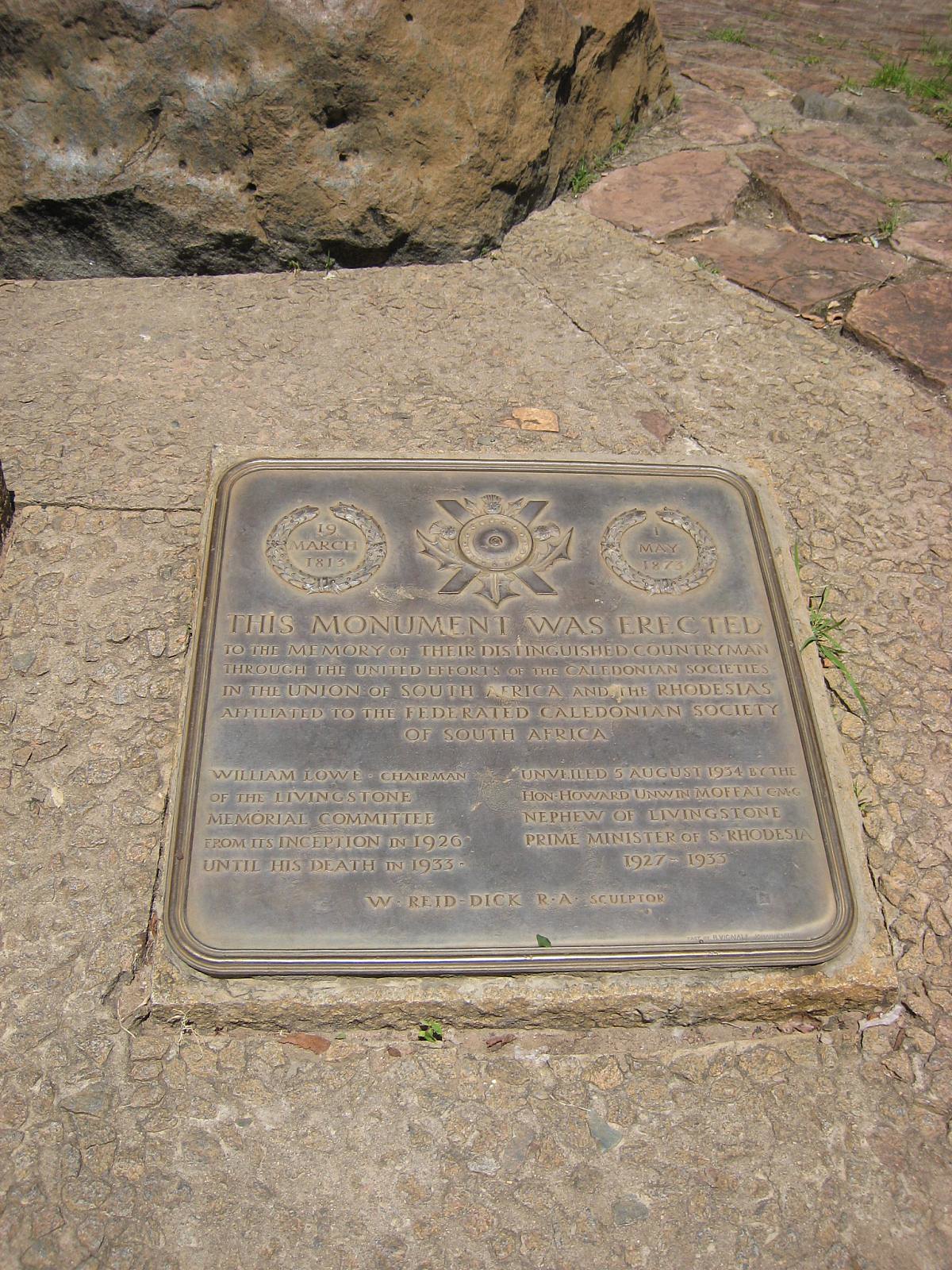A plaque set into a ground covered with brown rocks commemorates distinguished countrymen through the united efforts of the Caledonian Societies in the Union of South Africa and Rhodesia, affiliated with the Federated Caledonian Society of South Africa. The black metal plaque bears three symbols at the top and reads: "This monument was erected to the memory of their distinguished countrymen through the united efforts of the Caledonian Societies in the Union of South Africa and Rhodesia, affiliated to the Federal Caledonian Society of South Africa." Further text details that William Love served as chairman of the Livingstone Memorial Committee from its inception in 1926 until his death in 1935. It also notes that the plaque was unveiled on 5th August 1934 by Hon. Howard Unwin Moffat, nephew of Livingstone, Prime Minister of South Rhodesia from 1927 to 1933, and that W. Reid Dick, R.A., was the sculptor.